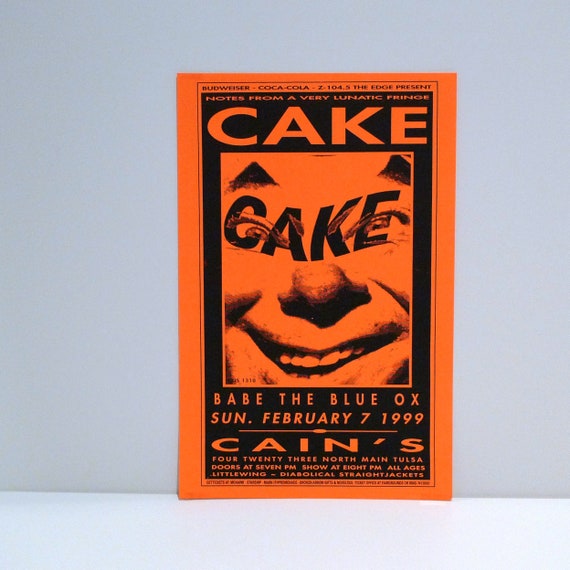The image is a vertical poster with an orange background framed by a black border. Dominating the center of the poster is a black-and-white depiction of a grinning clown's face with triangular eyebrows. The word "CAKE" is prominently written over the clown's eyes in an undulating font. Below this image are several rows of text: the top lines read, "Babe the Blue Ox," and "Sunday, February 7th, 1999." Further down, the text reads "Cain's," followed by "423 North Main, Tulsa," detailing the event's location. The poster indicates that doors open at 7 p.m. with the show starting at 8 p.m., and that it's an all-ages event. Additional smaller text at the bottom includes "Little Wing," "Diabolical," and "Straight Jackets," likely referencing other performers or details related to the event. The overall layout is slightly off-center, tilted more to the right.